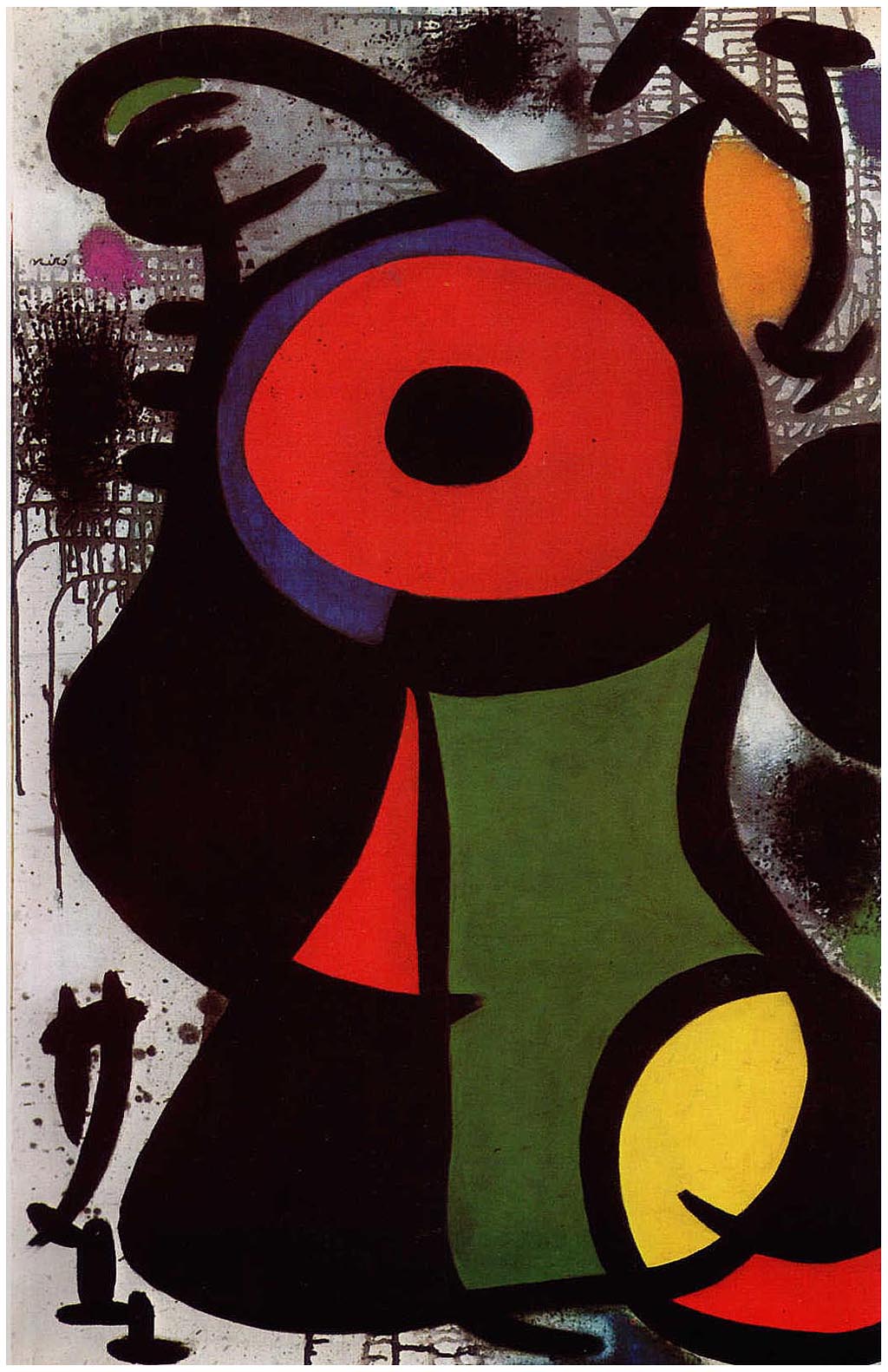This vertically aligned rectangular piece of abstract artwork features a predominantly gray background with splashes and splatters of black, most notably in the upper left and upper middle portions. In the upper middle area of the composition, there is a prominent red donut-shaped figure with a black center, evocative of an eye. Surrounding this central shape are various abstract forms and colors: black on the left, red in the middle, and a significant green area on the right that transitions into a small yellow section at the lower right corner.

Beneath the central red figure, the composition continues with more intriguing details. The left side features black shapes that resemble abstract symbols: two vertical lines with a horizontal line atop them, and two upside-down T shapes below. Additionally, there are black mounds and doodle-like scribbles below these symbols that add texture and complexity to the piece.

The artwork's abstract nature suggests a reconstructed portrait or figure, with elements such as the donut shape resembling an eye, and sections that could be interpreted as an ear or wing on the left, and another possibly yellow ear on the right. The lower portion of the image features an olive green section transitioning into yellow. The overall style is reminiscent of abstract expressionism, with its freeform lines and smudged, splattered background, enhanced by the unique blend of colors and symbols throughout the piece.